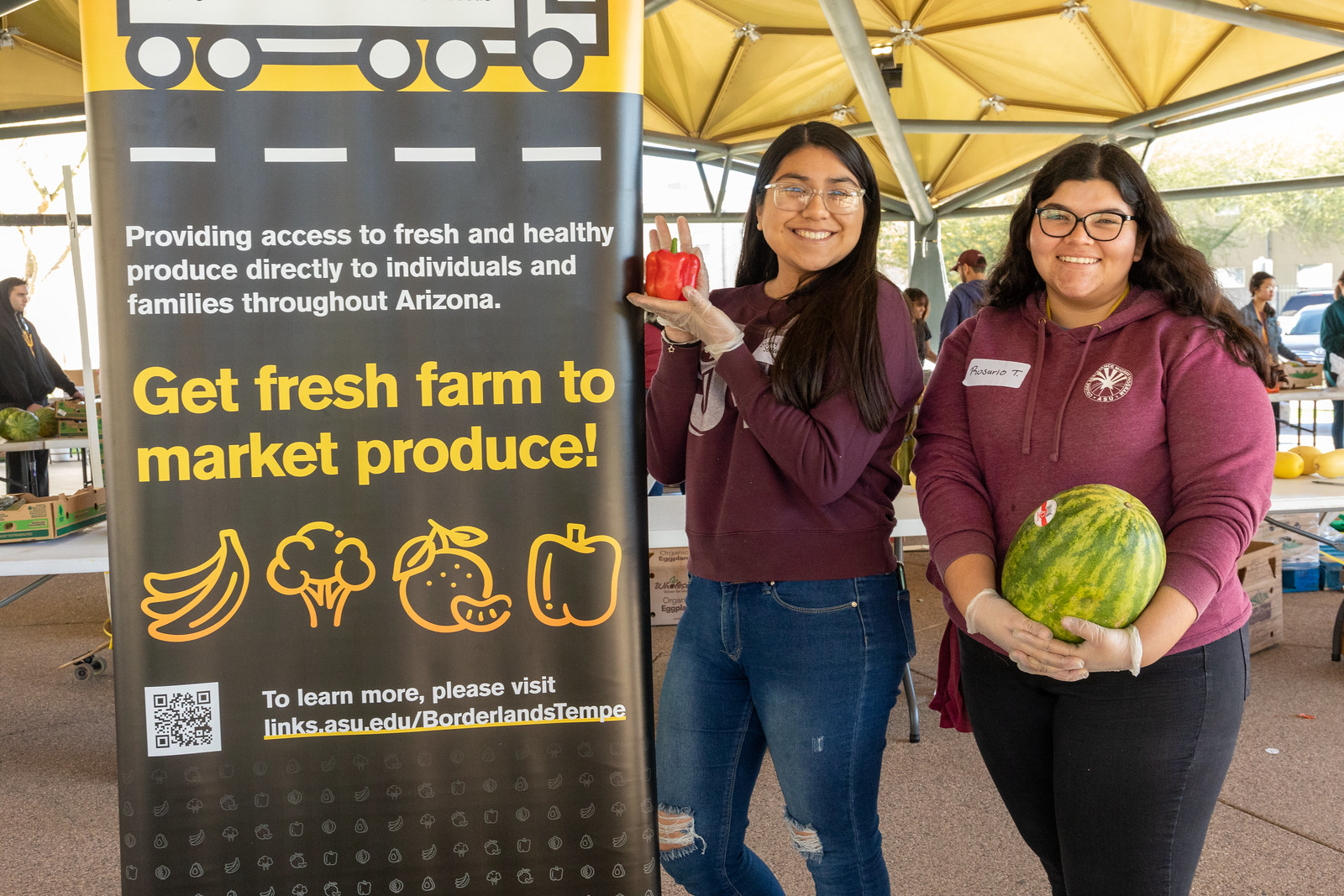In the image, two young Hispanic women stand beside a banner at what appears to be a farmer's market. Both women, wearing white plastic gloves, glasses, and red hoodies with jeans, are smiling warmly. The woman on the right, identified by her name tag as Rosario T., is holding a large watermelon, while the other woman is holding a red pepper. Although her name tag is obscured by her hair, she shares similar attire with Rosario: a red sweatshirt and glasses. 

Behind them, people are seated at tables with more fruits and vegetables visible, contributing to the market's bustling atmosphere. The banner they're standing next to reads, "Providing access to fresh and healthy produce directly to individuals and families throughout Arizona" in white lettering. Below this message, in yellow lettering, it states, "Get fresh farm to market produce." The banner includes images of bananas, broccoli, apples, and peppers, along with a QR code and a URL: links.asu.edu/borderlands-tempe. The image captures a moment of community service as these women contribute to distributing fresh produce.